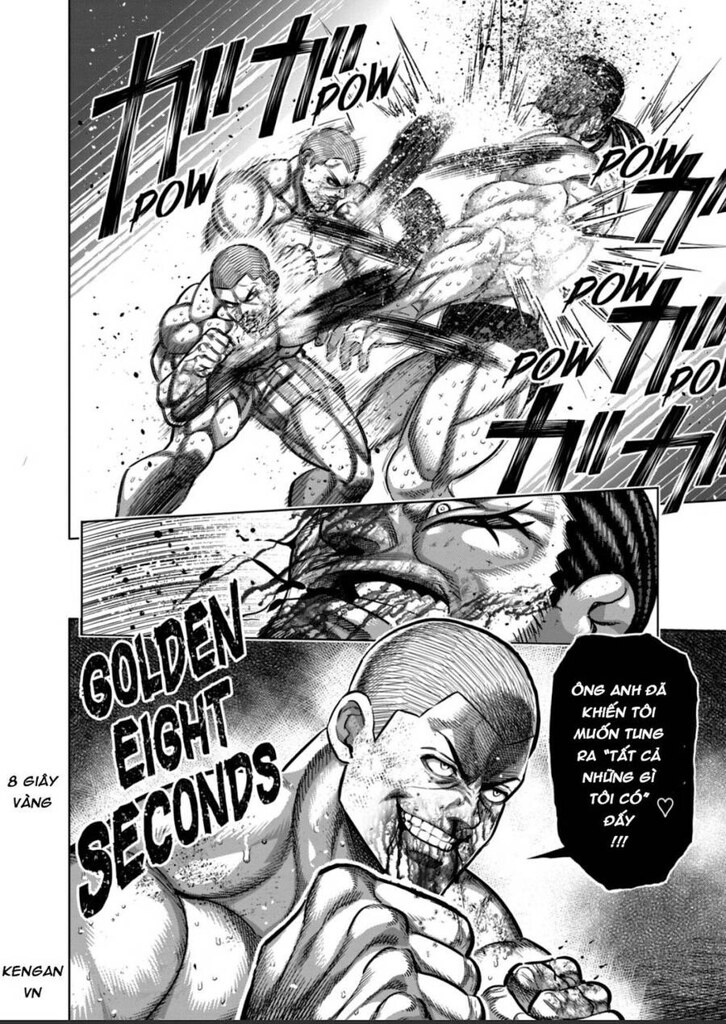The black-and-white comic strip consists of three panels, likely from a manga, illustrating an intense battle scene. In the first panel, a muscular fighter, on the left, repeatedly punches a much larger opponent, accompanied by sound effects like "Pow," "Till," and "Pow" scattered across the panel in both English and possibly Asian characters. The second, thinner panel captures the larger opponent's pained reaction, with blood dripping from his nose and his face contorted in agony. In the final panel, the determined and bloody-faced victor, the same muscular boxer from the first panel, stands with his fist raised. A speech bubble contains foreign text, while nearby English text reads "Golden 8 seconds," possibly indicating a significant moment in the fight. Other text, such as "A Guys Vans" and "Kengan VN," also appears in the lower-left corner, suggesting context or authorship in a foreign language.